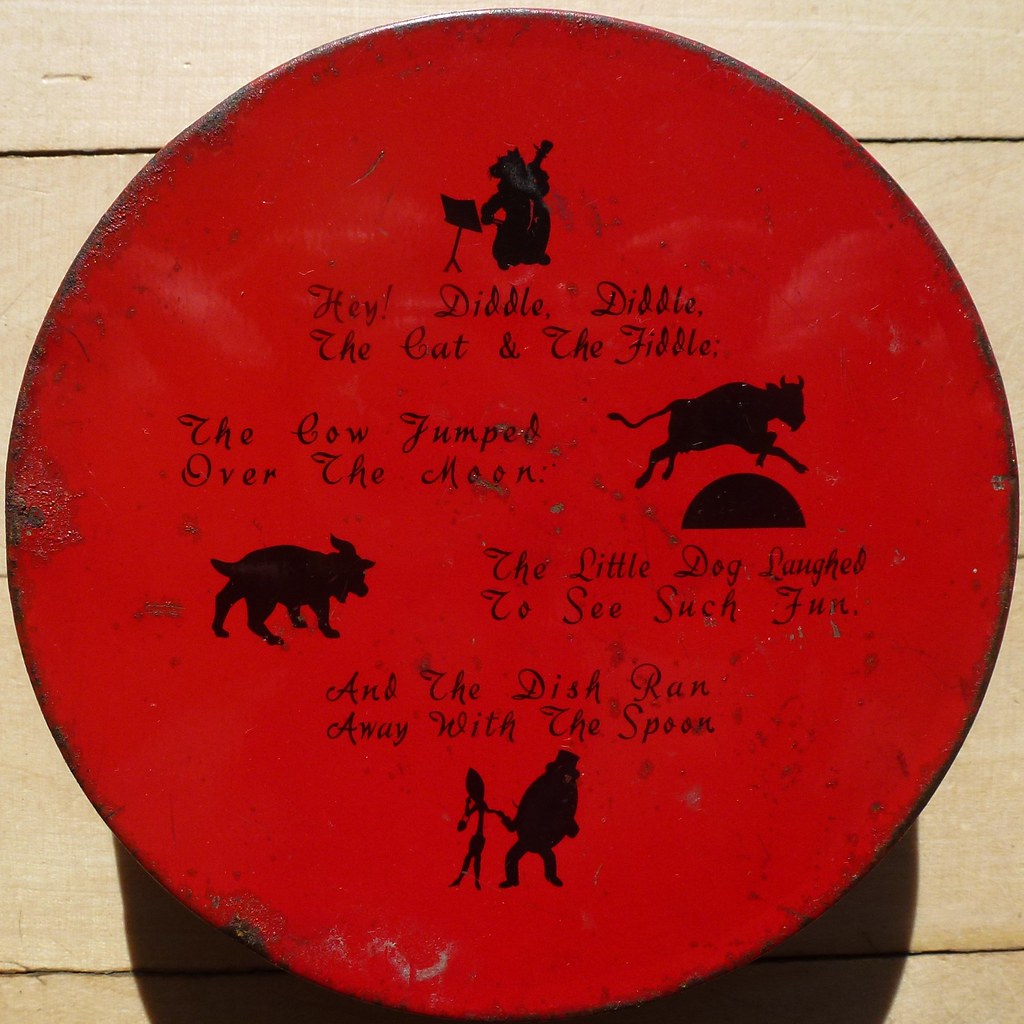The image showcases a vintage, red circular decorative piece, likely hanging on a wall in a household setting. The piece is set against an off-white background and is positioned on a light-colored wooden slatted surface, casting a soft shadow. It features the whimsical nursery rhyme "Hey Diddle Diddle" written in playful, curly, calligraphy-like black font. The rhyme is segmented into four paragraphs, each accompanied by detailed black silhouette illustrations: a cat playing a fiddle with a music stand, a cow leaping over a moon, a little dog standing and laughing, and a dish running away hand-in-hand with a spoon. The overall effect is one of rustic charm, with each element meticulously aligned to create a cohesive and enchanting visual narrative.